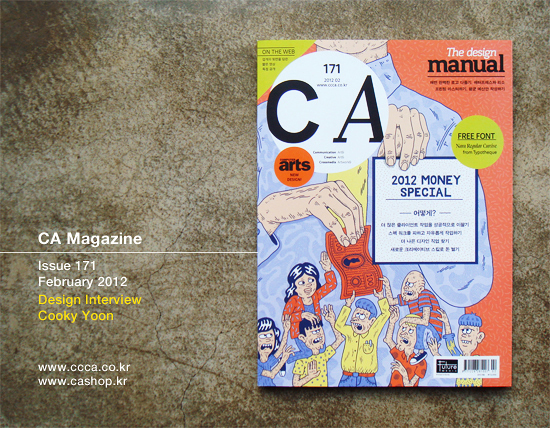This is a highly detailed and organized caption for the provided image:

**Cover of CA Magazine, Issue 171, February 2012.**

Featured prominently on the cover is an article titled "Design Interview" with Cookie Yoon. Below this, the magazine lists two websites: coco.co.kr and cashop.kr. The cover is adorned with a central image depicting a person holding a dollar bill and a sign that reads "2012 Money Special." Surrounding this individual are several people in yellow and red shirts, all reaching for the bill. The left side of the cover is accented in red, highlighting sections such as "Free Font." At the bottom, there is a barcode, and the word "Future" is faintly visible near the area. The magazine itself is placed on a stone-like surface, giving it a textured backdrop.